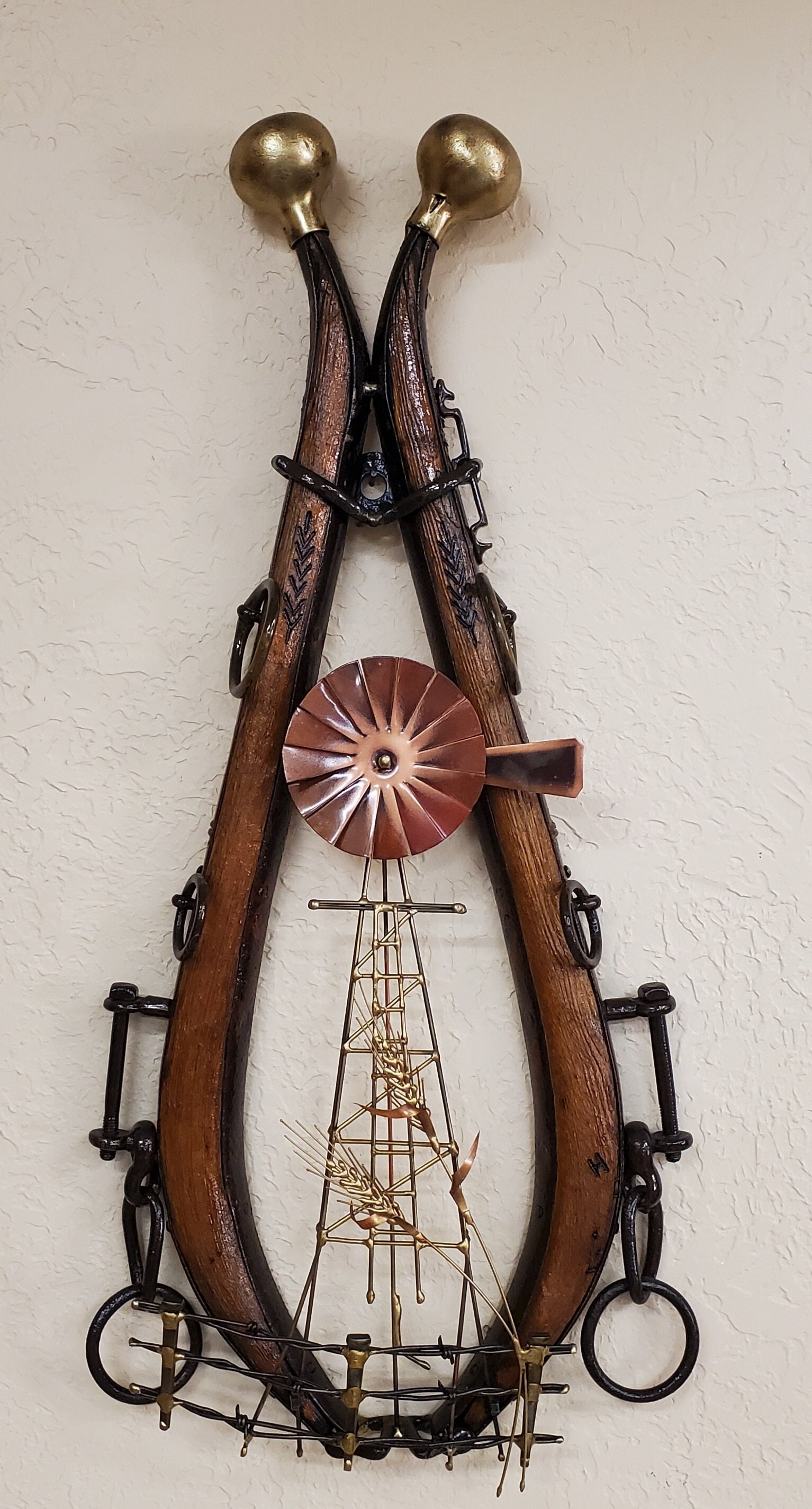The image depicts a close-up of a finely crafted wooden object, primarily composed of dark brown, hazelnut-colored wood with a teardrop-like shape that broadens slightly toward the top. The ellipsoid structure is intricately adorned with both metallic and wooden elements. At the top, where the teardrop shape begins to widen, there is a detailed, fan-like circular component fashioned from either brass or copper, resembling a windmill. Flanking this metal fan are two large brass balls that act as caps, adding a touch of elegance. The wooden sides are embellished with carved symbols of wheat, repeated multiple times, some of which are highlighted in gold. Several golden and wrought iron strings extend from the circular metal piece down towards the bottom, intertwining with metal strings and wrought iron rings, which provide additional support and decoration. Handles and smaller rings made from wrought iron, painted black, are affixed along the sides, completing this unique and artistic composition.